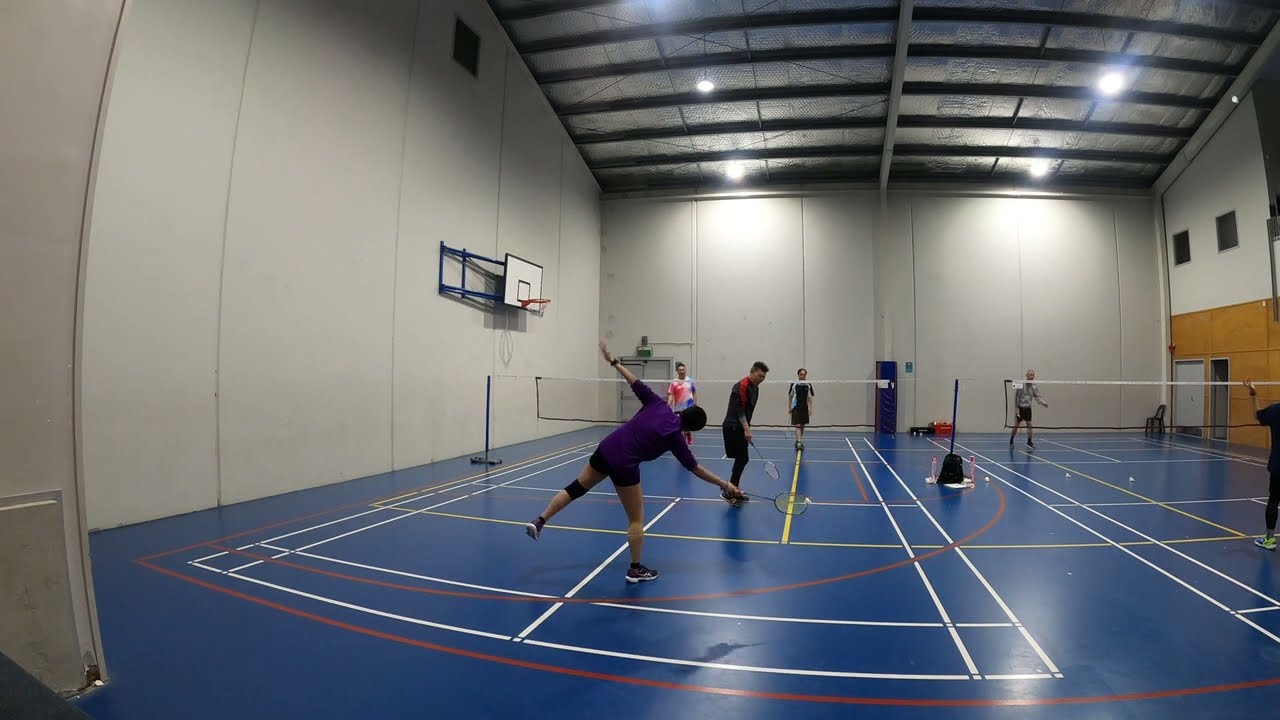This detailed image captures the inside of an illuminated gymnasium where two separate badminton games are taking place on adjacent courts. The floor is a dark blue, marked with white boundary lines and additional red and yellow lines indicating various play areas. On the left court, a doubles match is in progress featuring a woman in a purple shirt and black shorts, poised to strike, with her partner positioned ahead of her and their opponents on the opposite side. On the right court, a singles match is ongoing, with one player partially out of view and their opponent clearly visible across the net. The space features high walls with visible insulation and black beams supporting a ceiling outfitted with bright white lights. A basketball hoop is affixed to the left-hand wall, and two windows are visible on the far right wall, divided into white and golden sections.